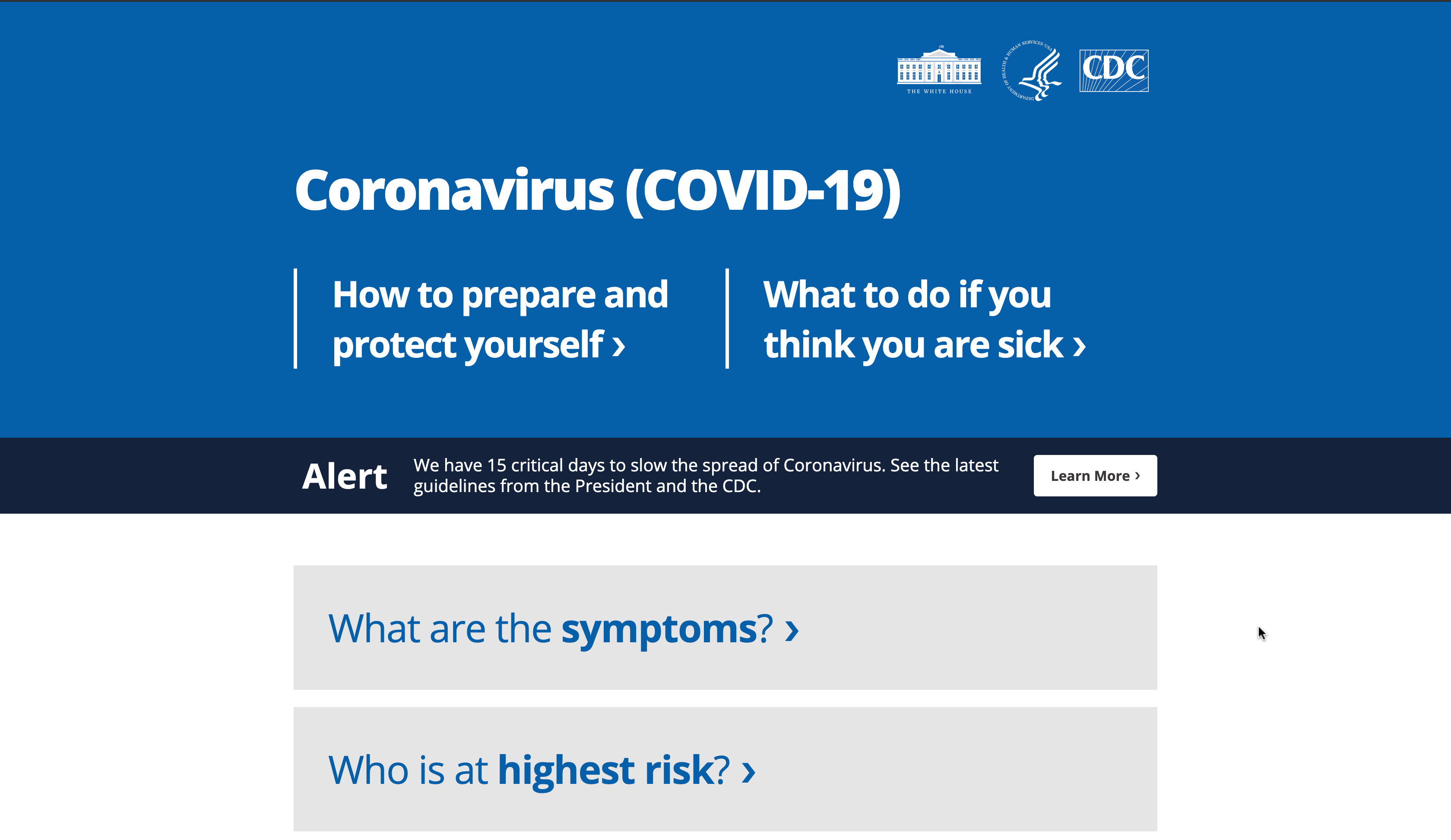This image is a cropped partial screenshot from a COVID-19 information webpage. 

At the top, there is a prominent blue header that spans the width of the screen. The header contains the word "coronavirus" followed by "(COVID-19)" in large white letters. Beneath this header, the words "How to Prepare and Protect Yourself" and "What to Do If You Think You Are Sick" are displayed in large white letters, each accompanied by an arrow pointing to the right.

Below this section is a dark blue border featuring an "Alert" message in white text. The alert reads: "We have 15 critical days to slow the spread of coronavirus. See the latest guidelines from the President and the CDC." To the right of this message is a box labeled "Learn More."

Following the alert section, the background turns white. There are two gray boxes with text surrounded by blue arrows. The first box, located at the top, is labeled "What are the symptoms?" with an arrow pointing to the left. Below it is another gray box labeled "Who's at the highest risk?" also with an arrow pointing to the left. Both sets of text are in blue.

The entire composition is designed to provide crucial COVID-19 information clearly and effectively.